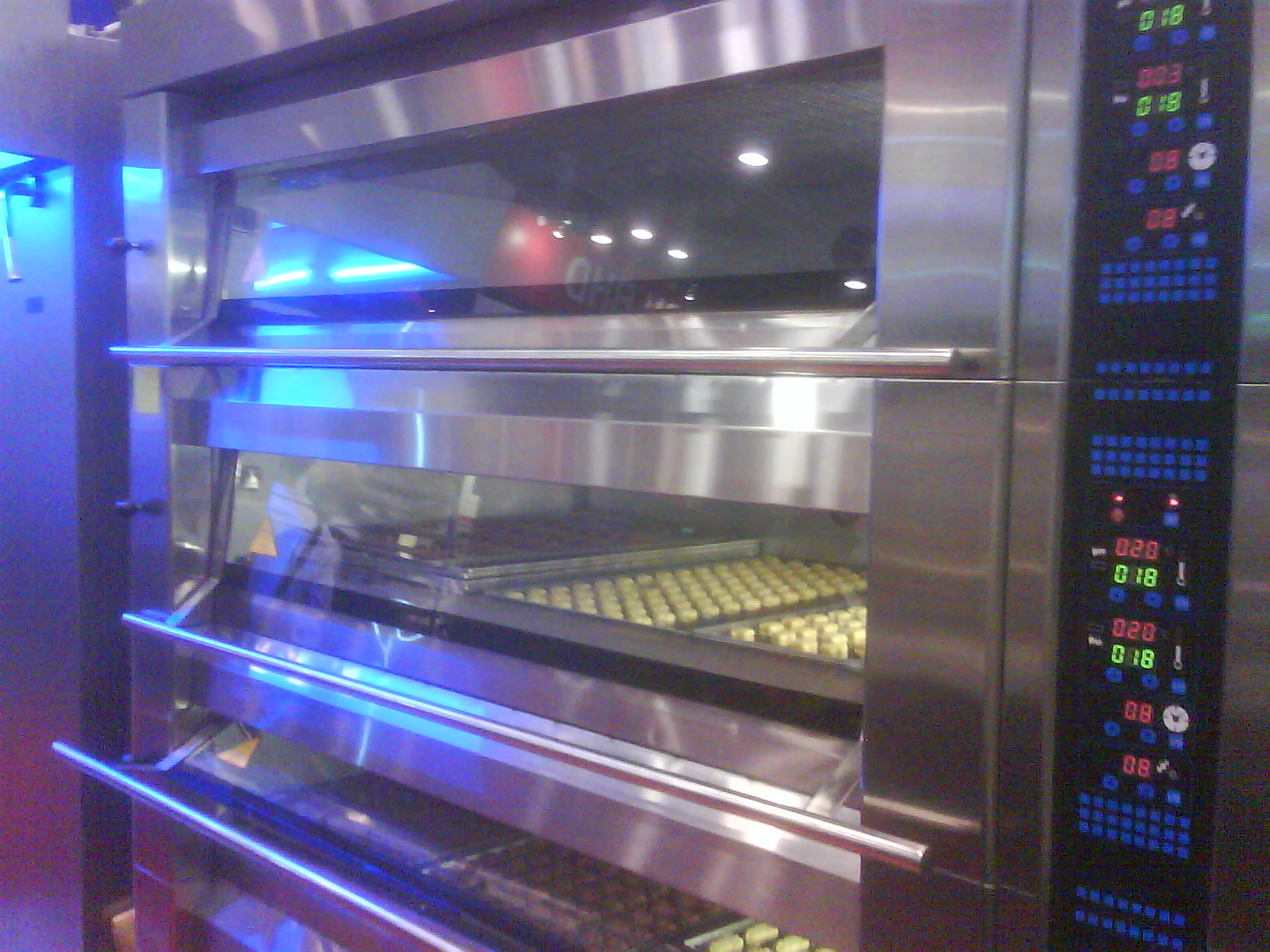The photograph depicts a blurred close-up of a large, high-tech industrial baking oven with multiple stacked compartments, often used in commercial kitchens or bakeries. The stainless steel unit stands roughly eight feet tall and features three separate glass-doored baking chambers, each illuminated by LED lights in blue, green, and red. The right side of the structure houses a sophisticated digital control panel with numerous buttons, LED displays, and temperature settings for each oven. Inside the two lower chambers, perfectly organized trays of pastries—resembling chocolates or small dough circles—are neatly lined up in grids. Each chamber contains three or four trays, with the pastries displaying a range of colors from beige to dark brown, suggesting different stages of baking or a variety of treats being prepared simultaneously. The reflective surfaces and diffuse lighting hint at an advanced, mechanized environment focused on precision baking.